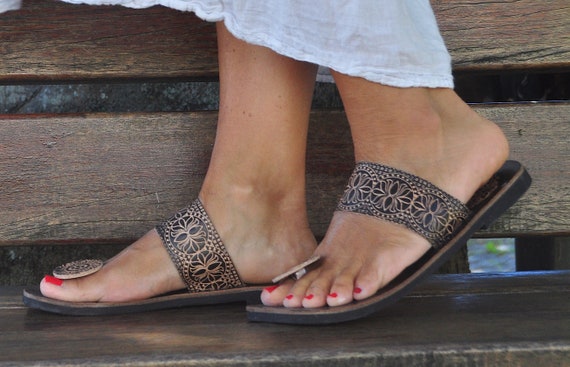This close-up image captures a woman's feet, showcasing her medium-toned, light brown skin and bright reddish-pink toenail polish. She is wearing elegant, dark brown open-toed sandals adorned with gold and black intricate patterns. The sandals feature a wide strap across the top and a smaller strap with a matching decorative disc between the big toe and the next toe, along with a tight yet ornate fit just in front of her ankle. She is standing on a park bench made of dark brown wood with visible slats, and the bottom of a flowing white dress or skirt is subtly visible above her ankles. No text is present in the image, emphasizing the focus on the footwear and setting.